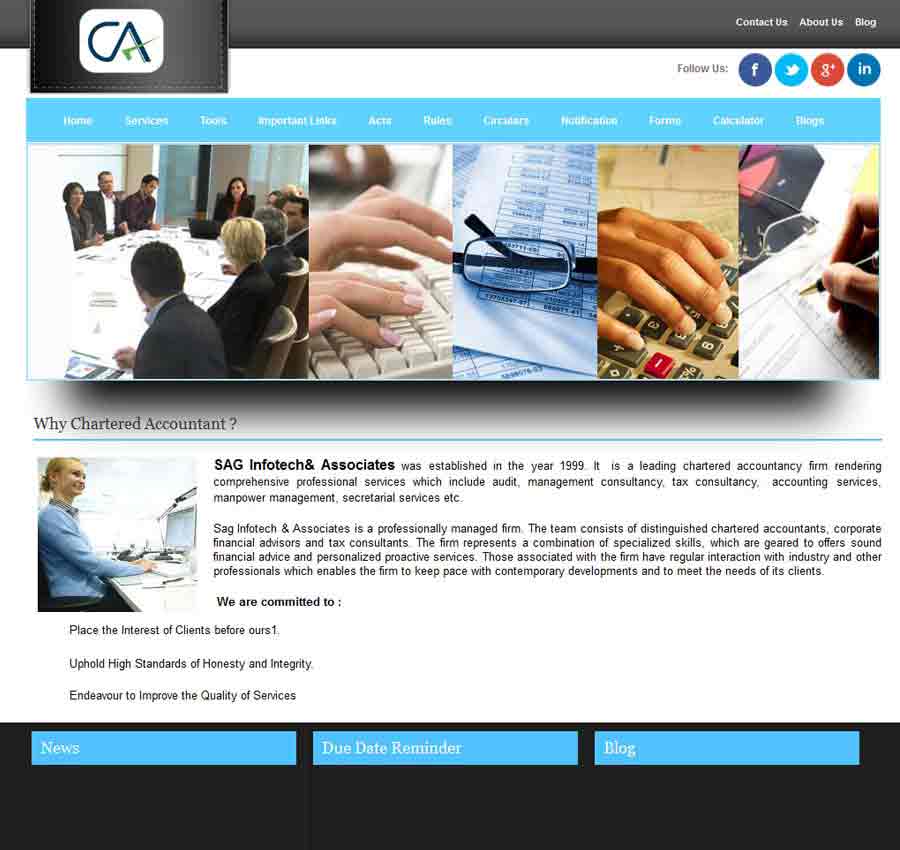At the top of the image, a dark gray bar spans across the width of the page. On the upper right, listed in white text, are the links "Contact Us," "About Us," and "Blog." On the left side, superimposed over the bar, is a long rectangular box featuring a white area with a blue-and-green logo. The logo appears to incorporate the letters "C" and "A" in blue, alongside a sideways-facing green checkmark.

Adjacent to this, on the right side, a white area contains the words "Follow Us" in black text, followed by social media logos for Facebook, Twitter (now known as X), Google Plus, and a blue circle with white text that says "I am." Below this section, a horizontal aqua blue bar presents menu options in white text, though they are somewhat difficult to read. From left to right, these options appear to be: Home, Services, Tours, Instagram, Links, Acts, something beginning with an "R," something beginning with a "C," Notifications, Forming, Calculator, and Blogs.

Beneath this menu, the image features a large, square picture on the left side showing several formally dressed individuals gathered around a table, seemingly engaged in a business meeting. Next to it, there are four tall rectangular images in a row. The first shows hands typing on a white keyboard. The second image displays part of a pair of glasses resting on some forms. The third reveals a hand typing on a calculator with papers visible above. The rightmost image depicts a pair of glasses on a table, with a hand holding a pen and filling out a form.

Just below this row of images, text in bold reads "Why Chartered Accountants," with a thin blue line underneath. Below this, another square image shows a Caucasian woman wearing a blue shirt, seated in front of a laptop in an office setting. Accompanying this image are two paragraphs of black text. The first paragraph features "SAG Infotech and Signed Associates" in bold at the beginning. The second paragraph ends with the bolded statement "we are committed to."

Further down, in black text, the image outlines several commitments: placing the interests of clients before their own, upholding high standards of honesty and integrity, and endeavoring to improve the quality of services.

At the very bottom, a large black text box includes three clickable aqua blue boxes with centered white text. The leftmost box says "News," the middle one says "Due Date Reminder," and the rightmost box says "Blog."